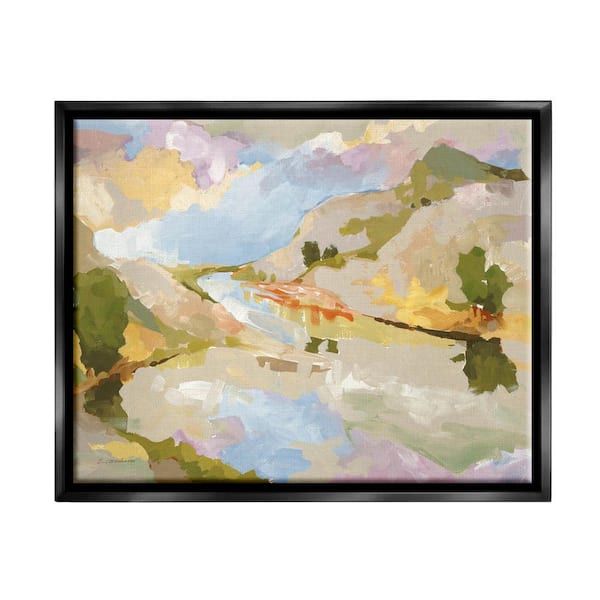This watercolor painting depicts a serene landscape featuring a meandering river flowing through snow-capped hills and mountains. The scene is characterized by contrasting colors and abstract impressions. The river originates from the upper center-left, curving gracefully through the landscape towards the bottom center-right, widening into a broad basin toward the lower center. Reflective and dynamic, the water mirrors hues of purple, yellow, and light blue, influenced by the vibrant sky above, which is a blend of blue, purple, yellow, and pink clouds suggesting the sun's glow.

The left shore transitions from green near the top to a blend of white sand and green near the bottom. Patches of greenery and reflections of plant leaves or clouds add richness to the scenery. On the right side, the shore exhibits an orangey middle section, bordered by yellow and softened by reflections of green trees.

The towering hills in the background showcase a mixed palette of army green, dark green, rust, and yellow, complementing the overall mystical and layered texture of the landscape. The interplay between land and sky creates a dreamy, almost surreal quality, with hints of an enigmatic town subtly integrated into the vista. This captivating composition captures the ethereal beauty of nature while blending elements of landscape and sky into a cohesive, flowing tableau.